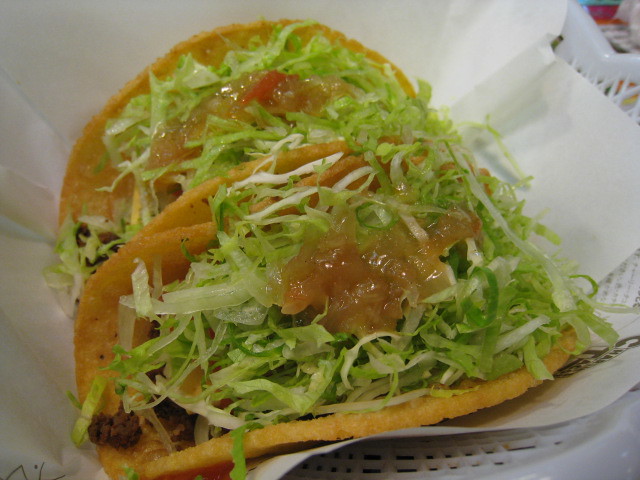The image is a close-up photograph of two mouthwatering street-style tacos, each nestled inside a white plastic basket lined with white tissue paper. The tacos, featuring crispy deep-fried yellow hard shells, look slightly soggy but inviting. They are packed with juicy ground beef that is peeking out from the bottoms, and are generously topped with finely shredded lettuce and possibly cabbage. Tiny pieces of cheese are sprinkled underneath an intriguing, orange-brown sauce that resembles a plum or marmalade topping. The two tacos are placed closely together, and to the right, a small container likely holding additional condiments can be seen, enhancing the inviting setup of this delectable dish.